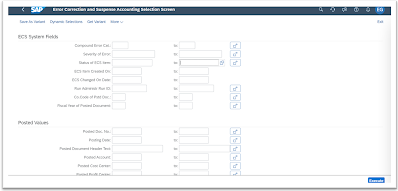The webpage features a minimalistic design dominated by a narrow blue border at the top, which contains five small icons. Below this, there's a section with blue text that is difficult to read due to its small size. 

The interface is organized into two main sections for data entry. The first section consists of two columns of vertical boxes, allowing for a total of 16 entries (8 per column). Below this, a thin line separates the second section, which permits 6 entries in two columns (three per column).

The page's layout is truncated at the bottom, where there is a distinctive white border. Finally, at the very bottom, there is an unmarked blue button. The functionality of this button is not specified due to its diminutive size making the text unreadable.